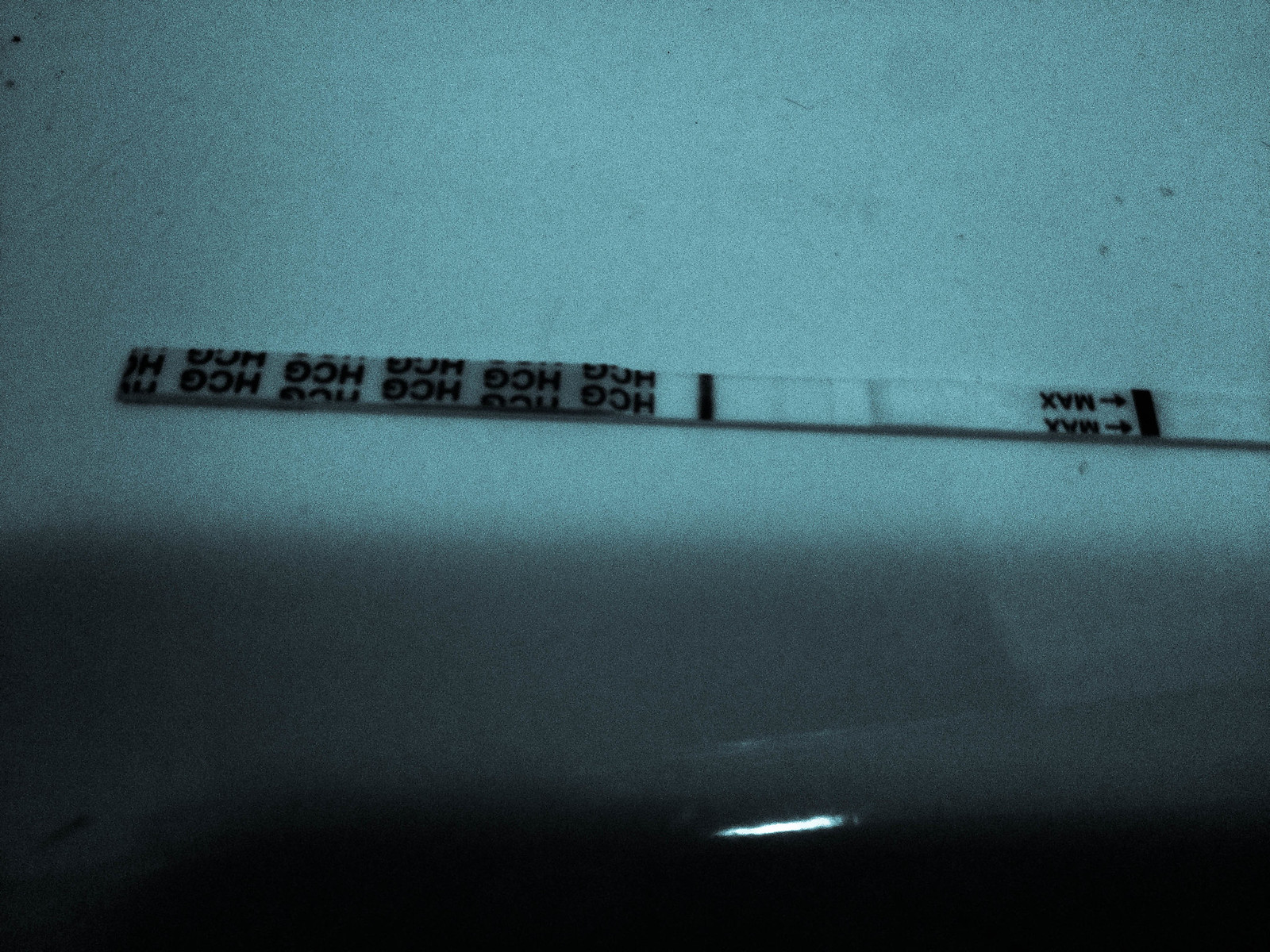In a dimly lit image, a pregnancy test is placed on a white countertop. The image is characterized by a pale blue light and a prominent shadow cast halfway up the frame. Central to the image is a strip extending from the right to the left, with clear, upside-down letters "hCG," indicating it is indeed a pregnancy test. On the far right of the strip, "max" is visible along with two arrows. Due to the poor lighting and shadow, it is difficult to determine if the test result is positive or negative. Additionally, a glare near the bottom center of the image adds an element of mystery, resembling a tear or imperfection on the tray holding the test, though the exact nature is obscured by the shadow.